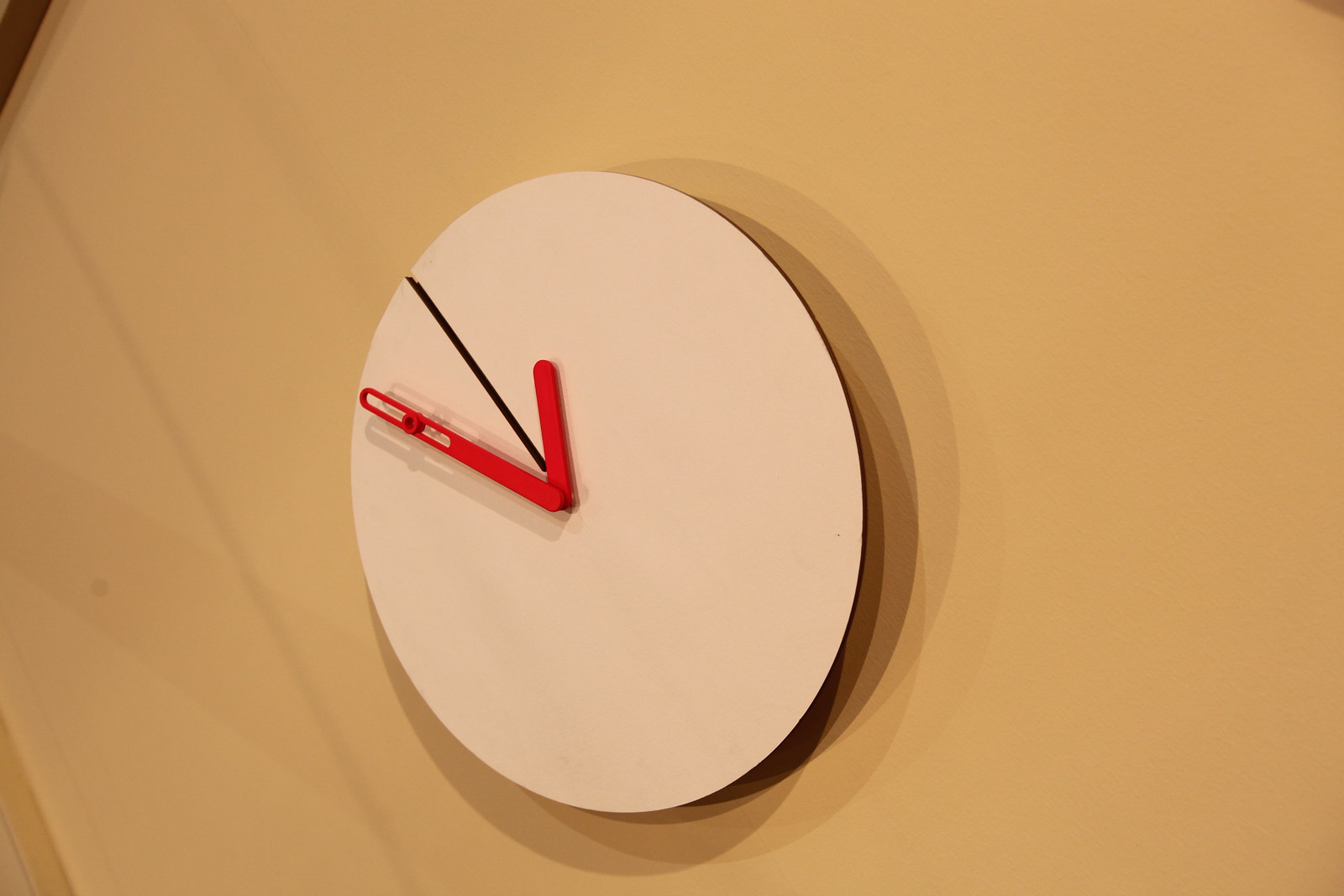The image features an unusual clock mounted on a peachy beige wall. The clock itself is a simple white circle with a minimalistic design. It appears to have a slight backing, giving it a subtle depth that keeps it from lying completely flat against the wall. The clock face is marked by a single black line extending from the center to the approximate position of the 10 on a traditional clock face. This black line is the only feature on the clock's surface apart from its hands. The clock has two red hands: a short, solid one and a longer one that has a small white label or an opening near its tip. Additionally, there is a small red button attached to the longer hand. The clock casts a shadow onto the white section behind it, adding a distinct visual element to its minimalist design.